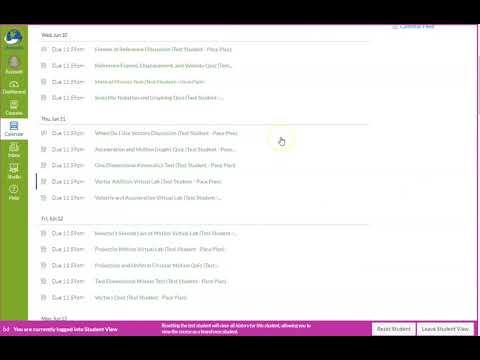This image displays a partial screenshot of a website, with significant portions obscured or cut off. At the very top, a black banner stretches across the width of the screen. Directly beneath it, on the left-hand side, there are remnants of text in a blue font, though the information is incomplete. A green border lines the left edge, embedded with various icons. The first icon is blue, and the subsequent icons are white, except for one that is highlighted and appears to open a secondary window within the interface.

The main body of the webpage reveals what seems to be a document, although the text is blurred, making it unreadable. On the left side of the document, there's a discernible title, separated from the rest of the text by a white horizontal line. Below this line, the content is divided into four sections of uniform length, each followed by sentences of varying lengths.

Further down, an additional section follows a similar format but includes one extra sub-section. A small marker line is visible next to this section, alongside what resembles a pointing finger icon near the center.

Continuing downward, there's a third section that mirrors the layout of the previous ones. Finally, at the very bottom of the image, a blue banner and a purple banner are visible, with two buttons positioned on the right-hand side of the purple banner.